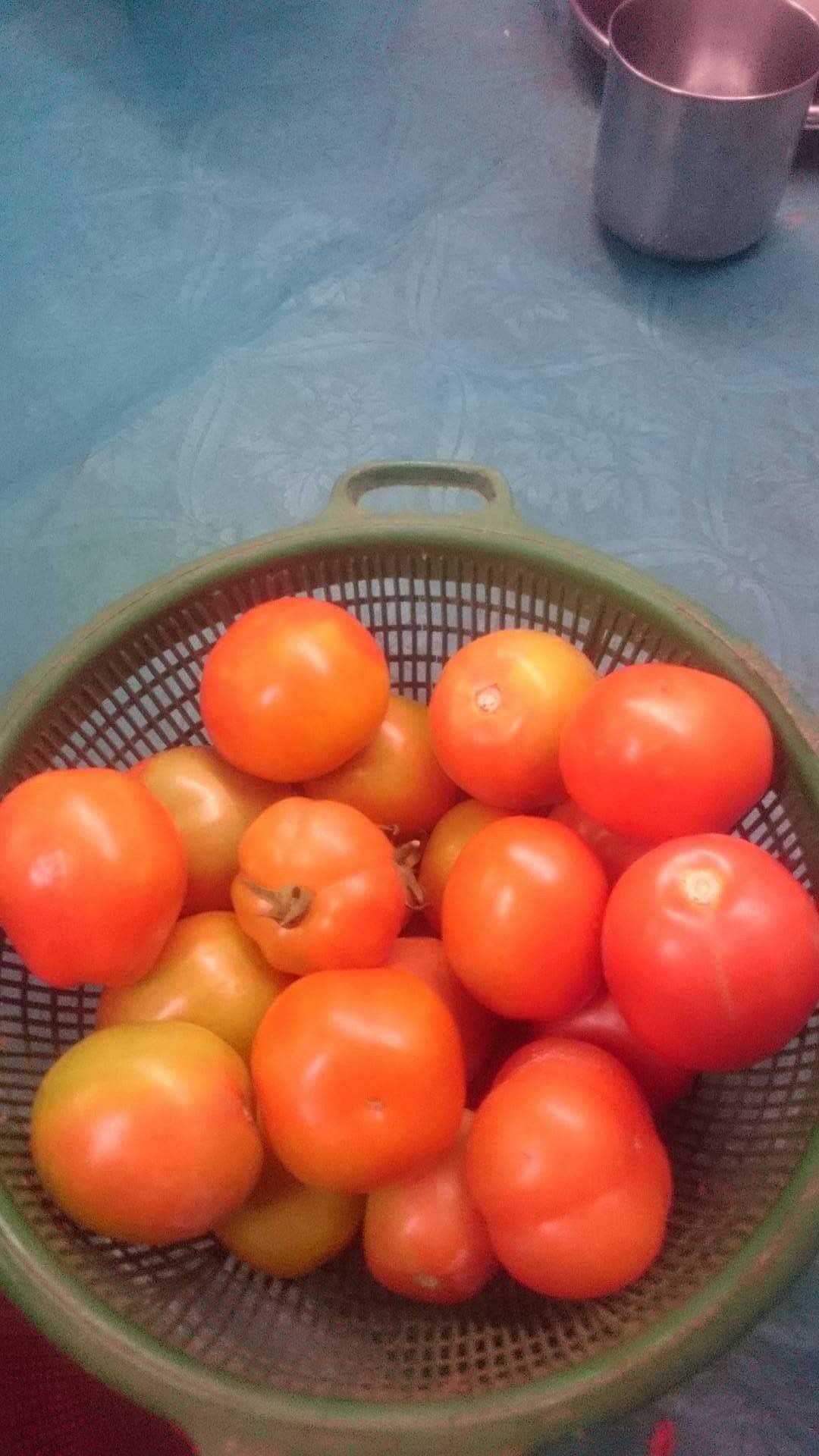An overhead photograph captures a vibrant scene centered around a green colander overflowing with tomatoes of various stages of ripeness, from luscious reds to shades of green and yellow. The colander, situated slightly off-center, showcases its distinctive hoop handle and fine square-shaped holes along its rim, which is notably dirty with a large patch of dirt prominently in the top right section. Inside the colander, approximately 18 tomatoes range in size from small to medium, and some still have their stems attached, displaying a palette of red, green, and even a blend of colors. This arrangement rests on a light blue tablecloth adorned with faint, almost imperceptible floral patterns that stretch diagonally across the frame. In the top right corner, a partial view of a silver cup adds a touch of metallic contrast to the rustic, earthy tones of the tomatoes and colander. The overall composition draws the eye to the rich, varied textures and colors, set against the subtle, patterned backdrop.